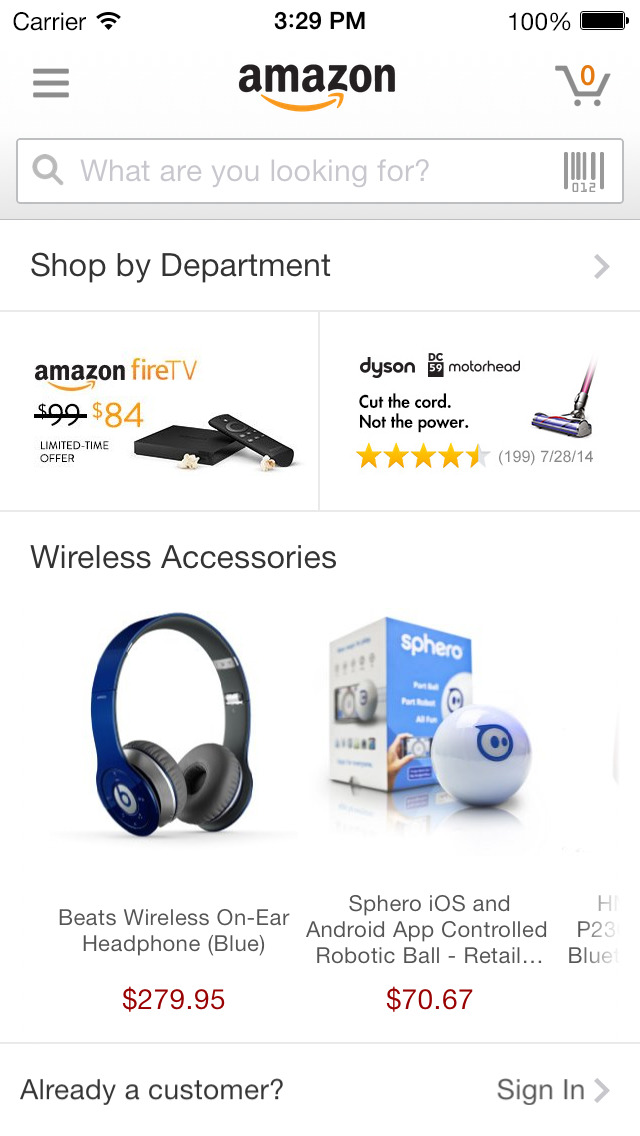The image appears to be a screenshot from a phone displaying the Amazon app interface. 

In the top left corner, it shows the word "Carrier," followed by a full signal bar and the time "3:29 p.m." Next to the time, the battery icon indicates a 100% charge, all in black.

Below this status bar, the left side features three small, gray horizontal lines. In the center, the Amazon logo is prominently displayed in black with a distinctive golden arrow connecting the letters "A" to "Z". To the right of the logo, there is a gray shopping cart icon with a golden zero inside it.

Beneath the logo, a white search bar invites users with the text "What are you looking for," accompanied by a small gray barcode icon.

Following the search bar, the text "Shop by Department" is displayed in black with a small gray arrow on the far right. A horizontal divider line separates sections within the app interface.

On the left side of the next section, "Amazon Fire TV" is listed, with the original price of $99.00 crossed out, and a current price of $84.00 displayed in orange, alongside the label "Limited Time Offer."

To the right, the "Dyson Motorhead" product is featured with the tagline "Cut the cord, not the power," and a rating of four and a half stars.

Below this, in a section labeled "Wireless Accessories," "Beats Wireless On-Ear Headphone" in blue are listed for $279.95, and "Sphero iOS and Android App-Controlled Robotic Ball" is priced at $70.67. Both prices are shown in red.

At the bottom of the screen, a prompt reads, "Already a customer? Sign in," with a line directing to the right.